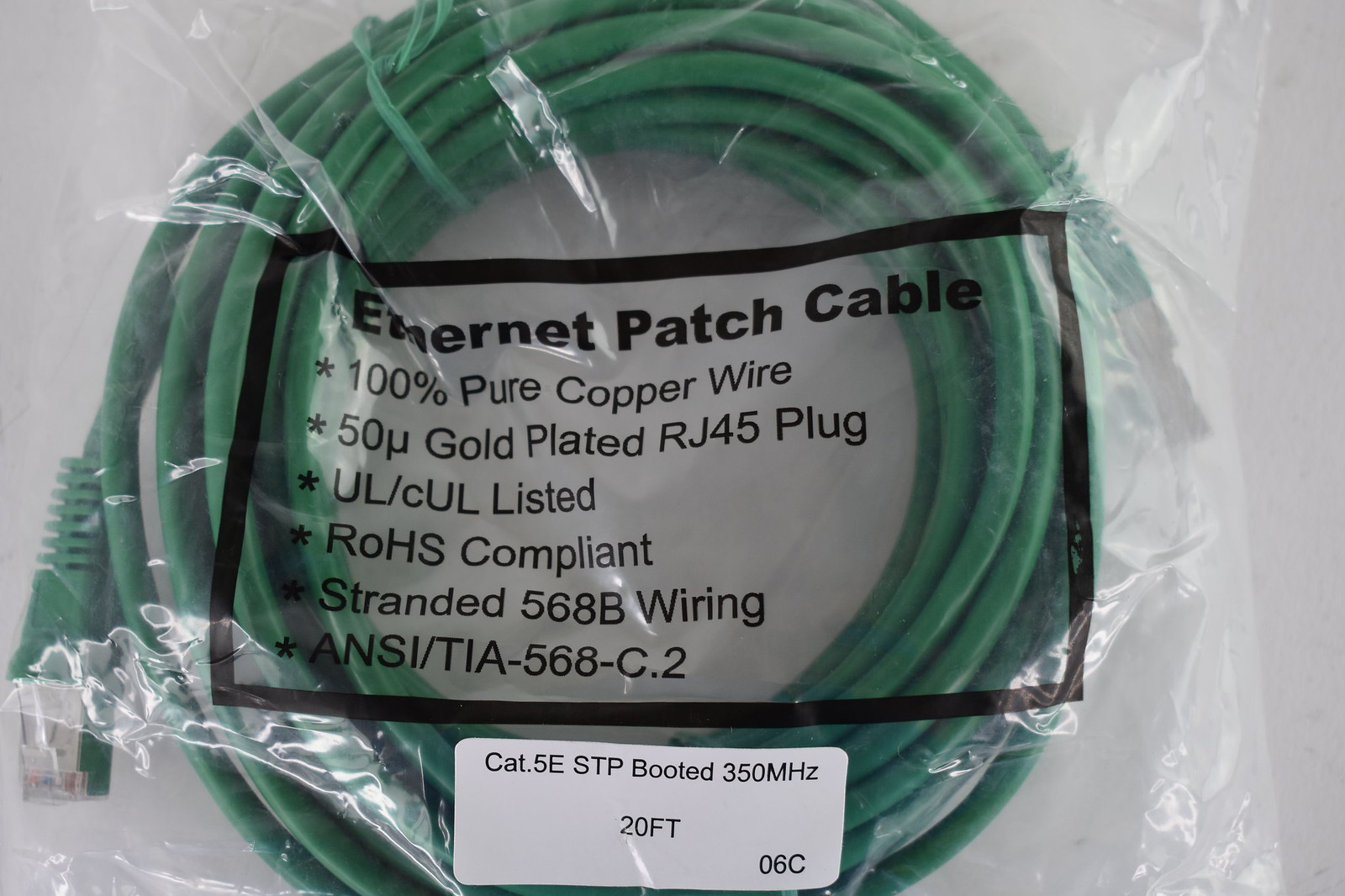This image shows a green Ethernet patch cable neatly coiled and packed in its original transparent plastic packaging. The front of the packaging features detailed specifications in black text inside a rectangular box. The text reads: "Ethernet patch cable, 100% pure copper wire, 50U gold-plated RJ45 plug, UL/CUL listed, ROHS compliant, stranded 568B wiring, ANSI/TIA-568-C.2". Beneath this rectangular box, a white sticker is affixed to the plastic bag, indicating additional details: "CAT.5E STP booted, 350 MHZ, 20 FT, 06C". The cable's vibrant green color contrasts with the clear packaging, making the detailed technical specifications and labeling easily visible.